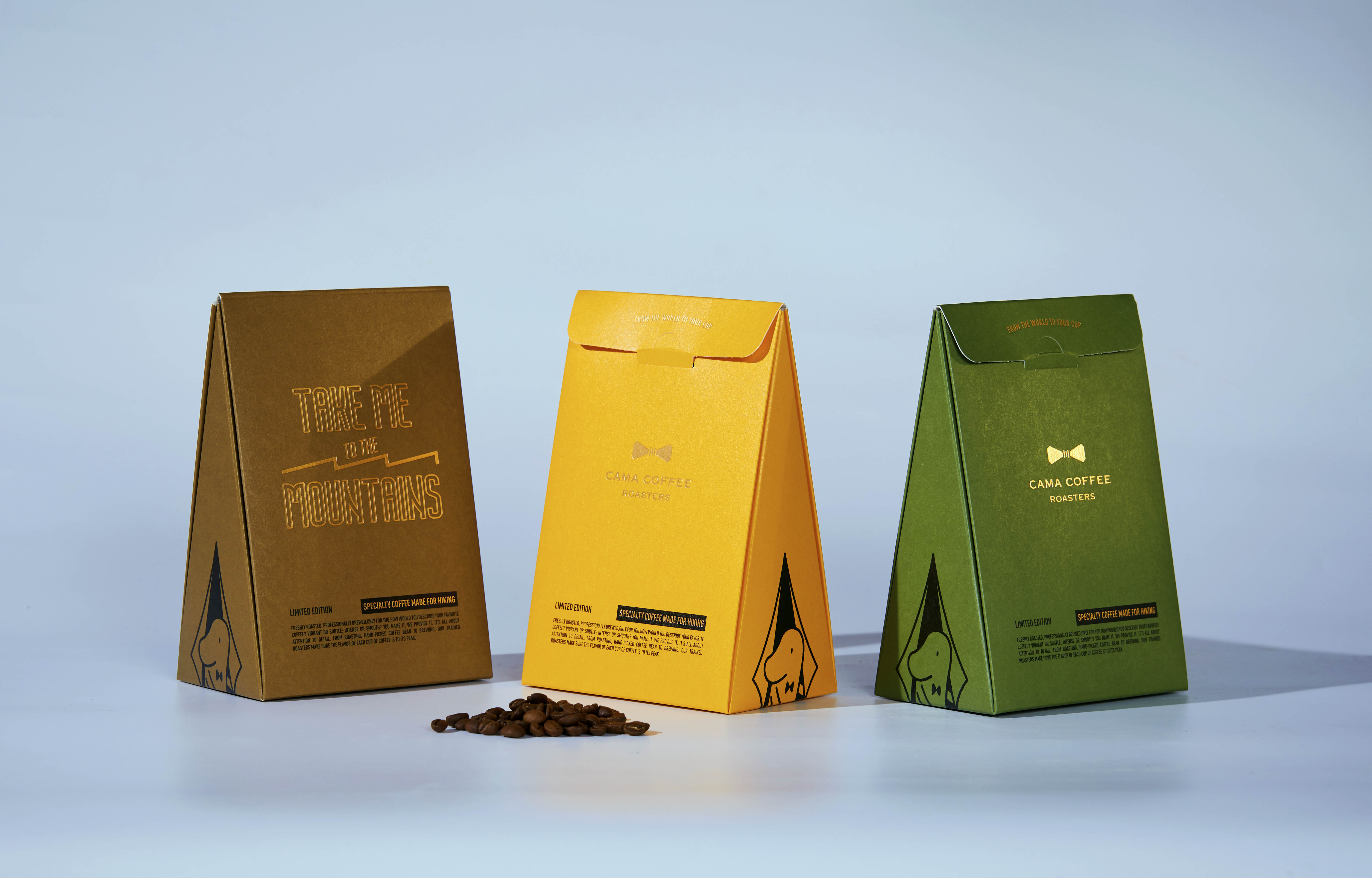Three neatly arranged bags of coffee beans are displayed side by side against a vibrant blue background. The first bag, on the left, is brown and triangular in shape, adorned with gold lettering that reads "Take me to the mountains." The middle bag, also triangular, is a bright yellow color and features the label "Canna Coffee." The final bag on the right is green, matching the shape of the others, with "Canna Coffee Roasters" elegantly inscribed in gold letters. In front of the brown and yellow bags, a small handful of coffee beans are scattered across the surface, adding a touch of rustic charm to the composition.